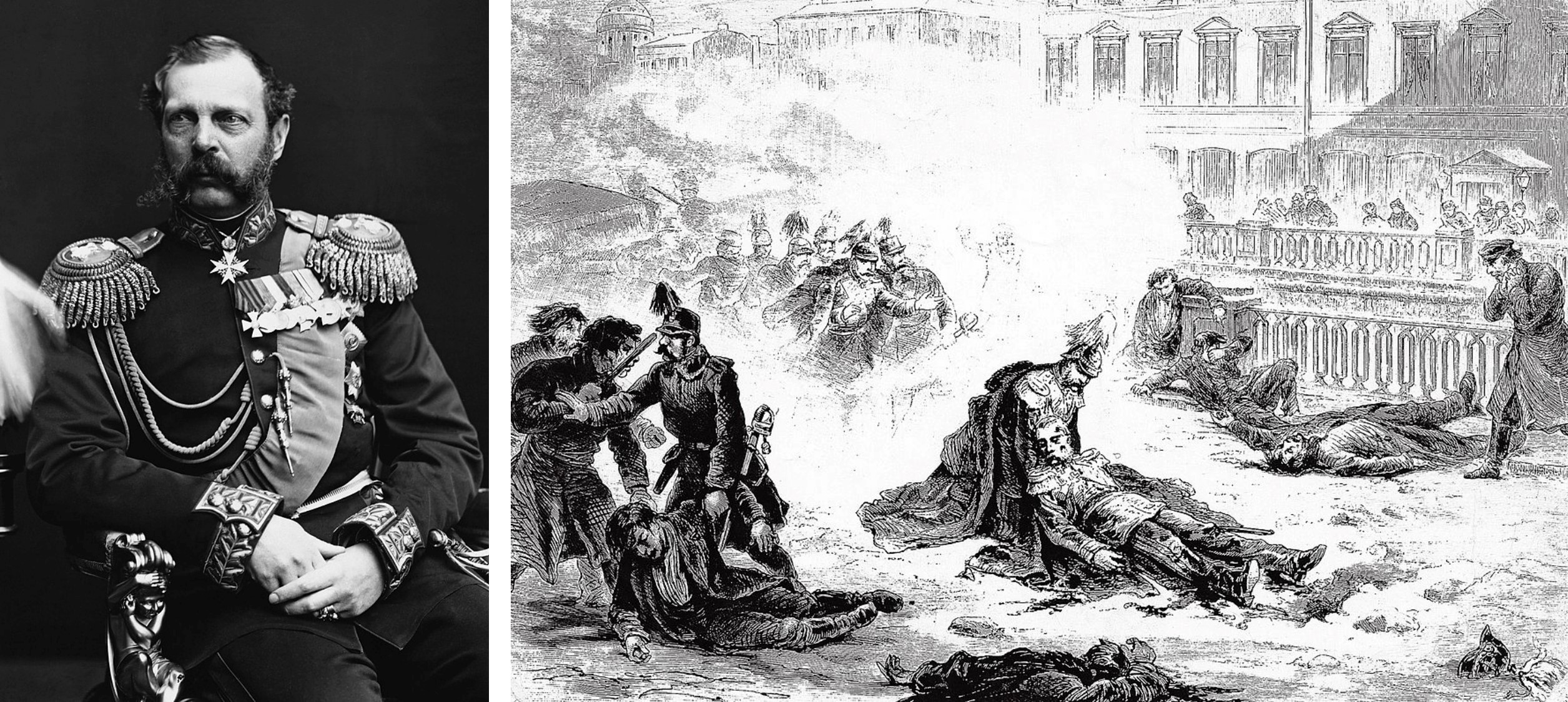This historical black-and-white illustration comprises two distinct yet interconnected images. On the left, a distinguished gentleman sits poised in an ornate chair characterized by golden adornments and an intricately designed armrest. Clad in a highly decorated military uniform, the man's attire features elaborate shoulder epaulettes with tassels, a cross medal draped from his collar, multiple medals across his left chest, chains from his right shoulder connected to his buttons, and gleaming cuffs at his sleeves. The background behind him is completely black, highlighting his solemn and authoritative presence. This individual, possibly a general or royalty, sports a short beard, balding head, and a prominent mustache.

On the right side, the scene dramatically shifts to a chaotic war reenactment depicted as a detailed pencil drawing. The battlefield is strewn with dead and dying figures, some of whom are being dragged off by others. Among the chaos, soldiers and civilians alike are captured in various states of distress — kneeling, attempting to rise, or frozen in shock and disbelief. In the midst of smoke and turmoil, a figure resembling the decorated man from the left image appears to lie lifeless or critically injured, further connecting the images. The background of this grim scene includes buildings shrouded in smoke, adding to the sense of devastation and urgency. This powerful juxtaposition captures both the valor and the human cost of warfare.